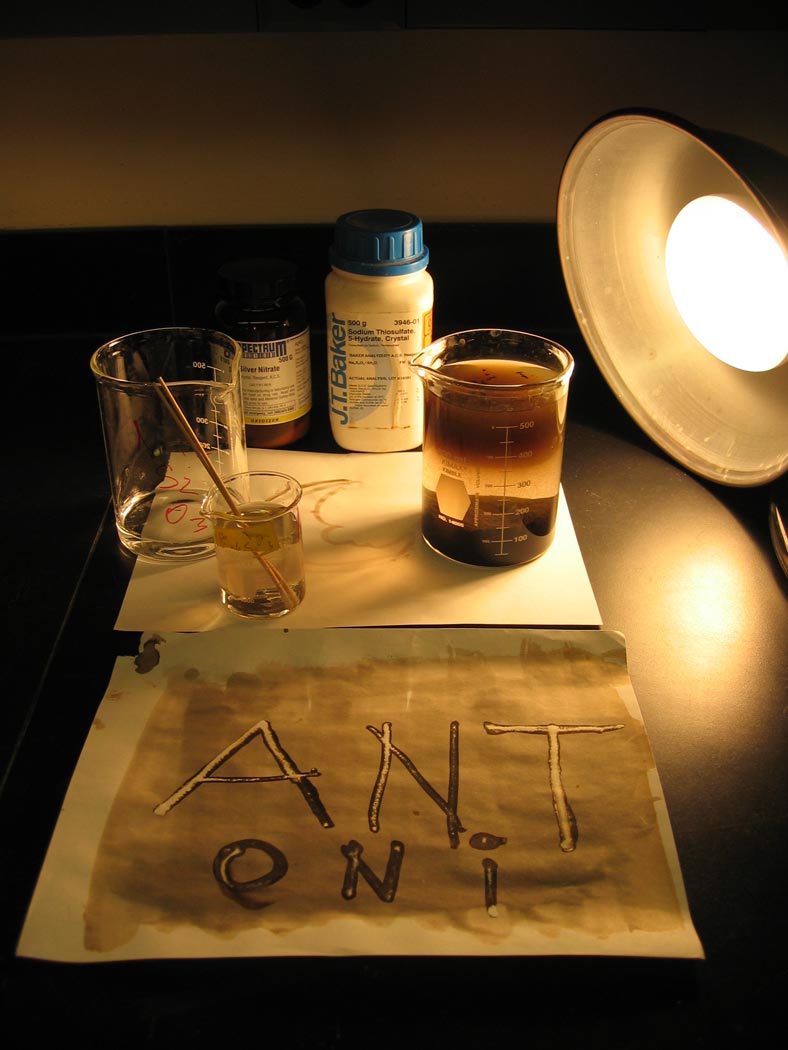The photograph features a scientific setup illuminated by a spotlight in the upper right corner. Central to the image are three glass beakers placed on a white surface. The beaker on the right contains a brown liquid, while the one on the left is empty, and a smaller beaker appears to have a straw in it. In the background, there are two containers: a white jar with a blue cap labeled "JT Baker" in blue text, and another plastic jar with a white label and a black top. In the foreground, there is a square napkin with a brown center, where the text "A-N-T" is written in large beige or brown letters, and below it in smaller letters, "O-N-I" or "Antony." The setup is accompanied by a lampshade and various scientific metrics printed on the beakers.